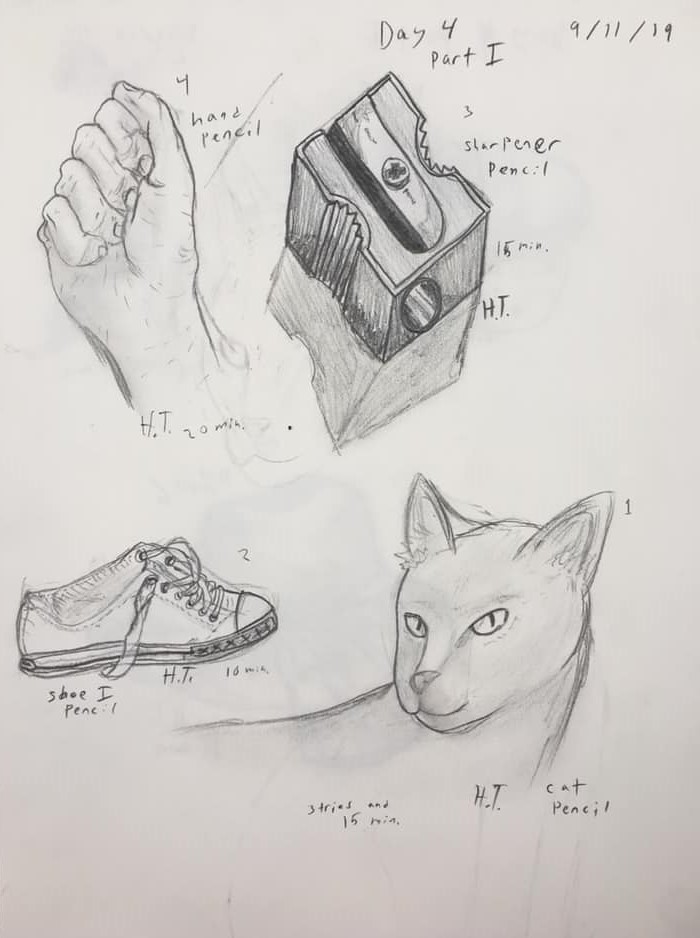The image features a scanned A4 sheet of white paper filled with detailed pencil sketches. Dated 9/11/19 in the upper right-hand corner, the sheet is labeled "Day 4, Part 1." The first sketch, positioned at the top-left, depicts a right hand from the wrist up making a clenched fist with the thumb on the outside. The drawing is marked "hand pencil" and noted to have taken "20 minutes" (H.T.). The hand sketch is highly detailed, showcasing precise crease lines and fingernails.

To the right of the hand is a meticulously drawn rectangular pencil sharpener, labeled "sharpener pencil 15 minutes H.T." The sharpener features an opening on the side, a screw on top, and noticeable indentations with a serrated edge, casting a shadow for added realism.

On the second row, there is a sketch of a sneaker with untied laces, labeled "shoe pencil HT 10 minutes." The shoe resembles a Converse sneaker, with detailed lacing and X-shaped patterns along the sides, emphasizing the textural elements.

The final drawing on the bottom right is of a cat's head and neck, giving the impression of a large feline, perhaps a leopard. Labeled "cat pencil 15 minutes HT," it displays pointed ears and a sly expression, with the cat looking back over its body, capturing the essence of the animal in a lifelike manner. All sketches are rendered in graphite pencil, showcasing the artist's practice and progress in drawing.